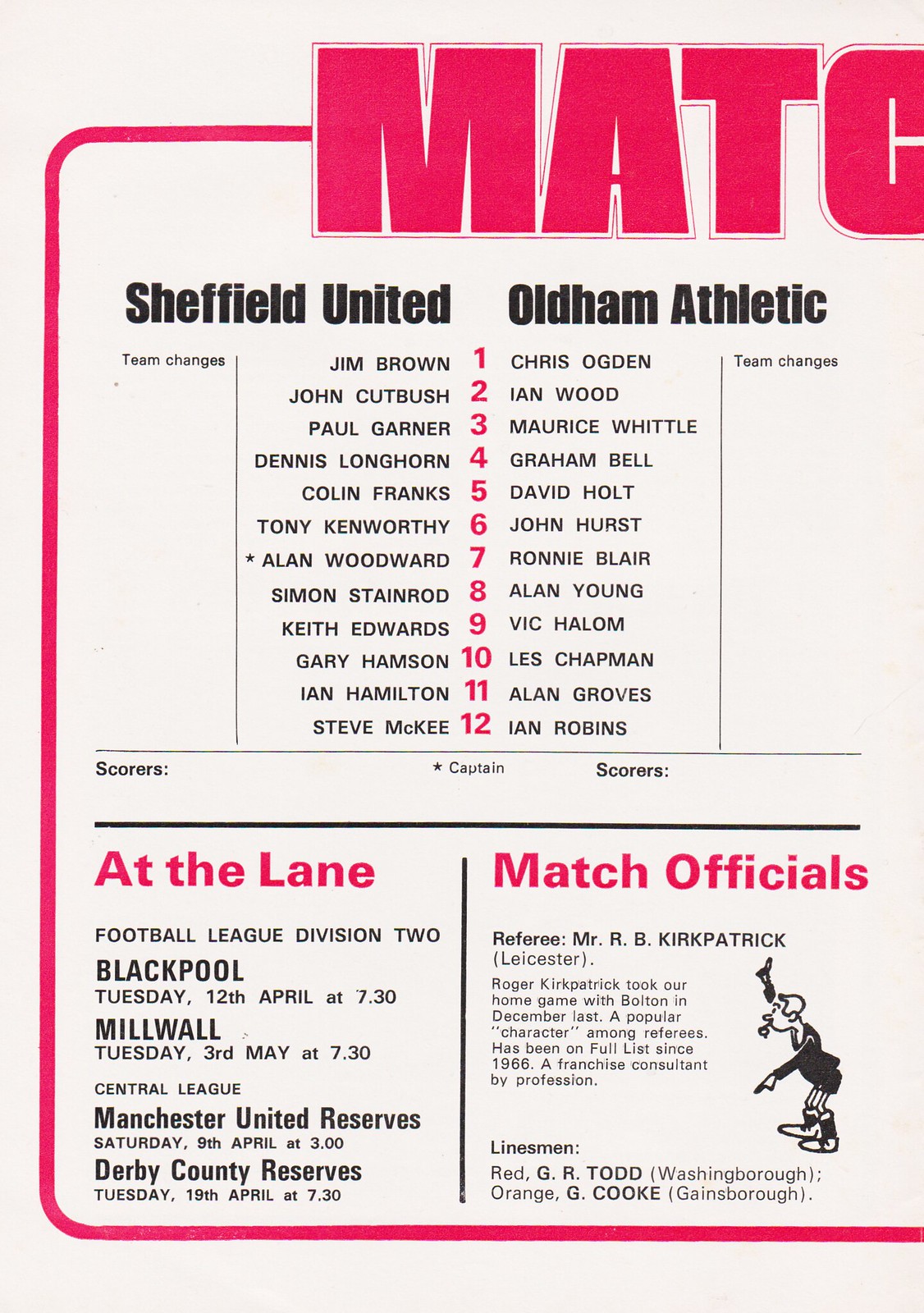This image captures a portion of a detailed sports poster related to English football. The white poster with red and black lettering is framed by a red border and is slightly cut off on the right side. At the top, the partially visible word "match" indicates the context, though it extends beyond the paper's edge. 

The main section is divided into two columns: on the left, it lists "Sheffield United Football Club" and their team members, and on the right, it lists "Oldham Athletic Football Club" and their team members. Below these listings, the content is further divided into two areas separated by a black line. 

On the left, under the heading "At the Lane" in bright red letters, it details upcoming fixtures for Sheffield United, including:
- Football League Division 2 match against Blackpool on Tuesday, April 12th at 7:30 PM
- Match against Millwall on Tuesday, May 3rd at 7:30 PM
- Central League match against Manchester United Reserves on Saturday, April 9th at 3:00 PM
- Derby County Reserves match on Tuesday, April 19th at 7:30 PM

On the right, under the bright red heading "Match Officials," it lists the officials overseeing the matches, and features a small drawing of a man with a whistle holding up his hand. The scores section beneath the team listings is blank, suggesting the poster is a blank copy meant to display upcoming matches and official details.